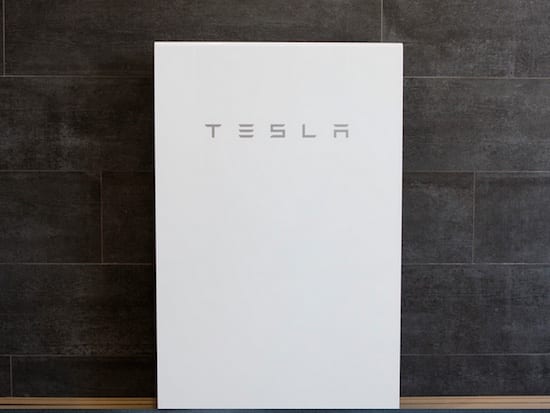The image features a wall composed of gray bricks, each brick exhibiting a subtle gradient that includes shades of gray, blue, and a hint of red, creating an intricate, multi-colored texture. Attached to the wall is a light gray, rectangular poster positioned vertically. The poster prominently displays the word "Tesla" in a unique, stylized font. The "T" is depicted as a conventional capital T, while the "E" consists of three vertical lines, omitting the horizontal line typically found in the letter. The "S" and "L" are in a standard font, and the "A" is creatively rendered as half of a square with a line above, resembling the upper portion of a square resting atop the vertical line.